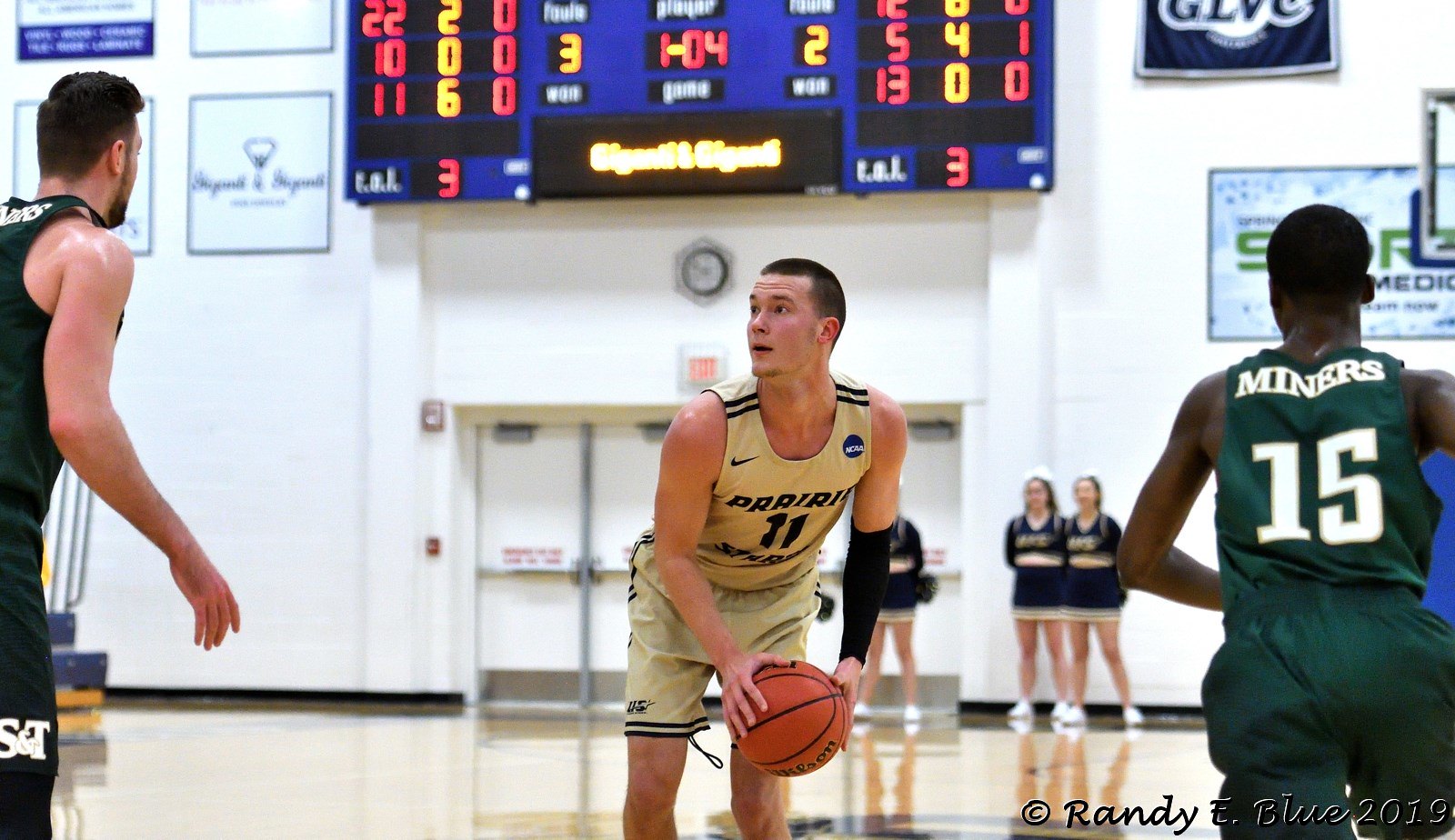This photograph captures an intense moment of a basketball game, likely at a high school or college level, taken from down on the court. Central to the image is a male player in a pale yellow jersey with black text, bearing the number 11 and partially reading "Perry." He stands poised with the basketball near his knees, gazing to his right towards a tall, cropped-out defender in black. On the right side of the frame, another opposing player, number 15, is clad in a dark green jersey with "Miners" inscribed in white and faces away from the viewer. The background reveals a typical gymnasium setting, featuring double doors and a big blue scoreboard displaying a score of 3-2 with 1:04 elapsed, in vibrant red and yellow numerics. Flanking the doors are three cheerleaders dressed in green and white, alongside multiple indistinct banners. The bottom right corner of the photo is marked with a copyright notice: "Randy E. Blue 2019," hinting at the photographer's identity.